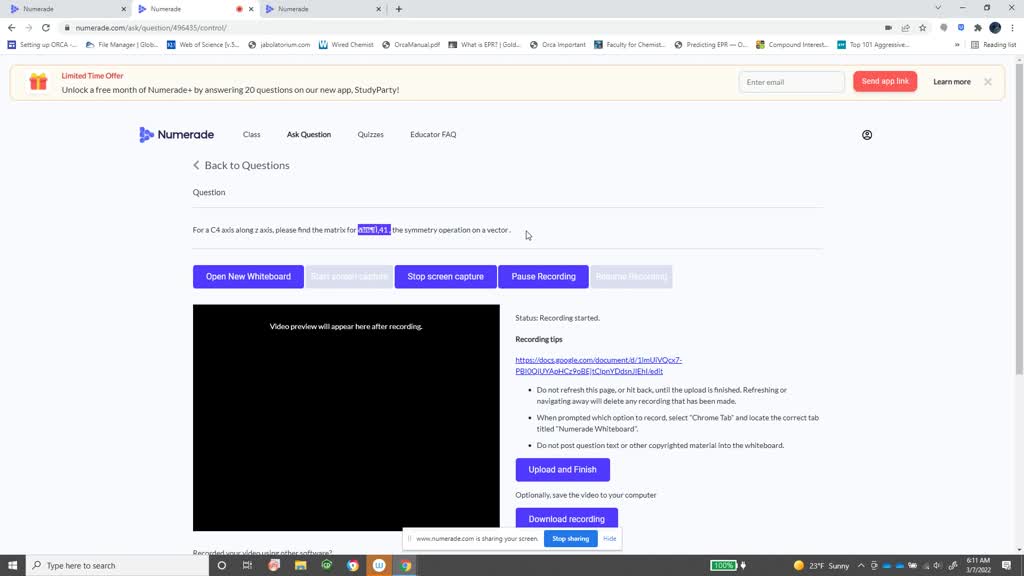This is a detailed caption for a landscape-oriented screenshot of the NumerAid website:

---

The image displays a landscape-oriented screenshot of the NumerAid website with three browser tabs open, all labeled "NumerAid." Despite the small font, some key elements are discernible. A prominent header on the active tab announces a limited-time offer: "Unlock a free month of NumerAid Plus by answering 20 questions on our new app, Study Party."

Below this header are several navigation options - NumerAid, CLASK, Ask Questions, Quizzes, Educator, and Facts. Another section seems to feature a complex question, potentially for a mathematical or programming operation: "For a C4 axis along the Z axis, please find the matrix for the Symmetry Operator on a Vector."

Along the interface, various options are available for interaction, including "Open new whiteboard," "Stop screen capture," "Poor recording," "Upload and finish," and "Download recording." A repeated voice command, "Alexa, Stop," indicates an interruption or distraction captured during the screenshot.

Additionally, a white bar at the top of the screen reads "Stop sharing," confirming that the screen was actively being shared with someone else. At the bottom right corner, a blue button labeled "Stop sharing" and another option to "Hide" the sharing indicator are visible.